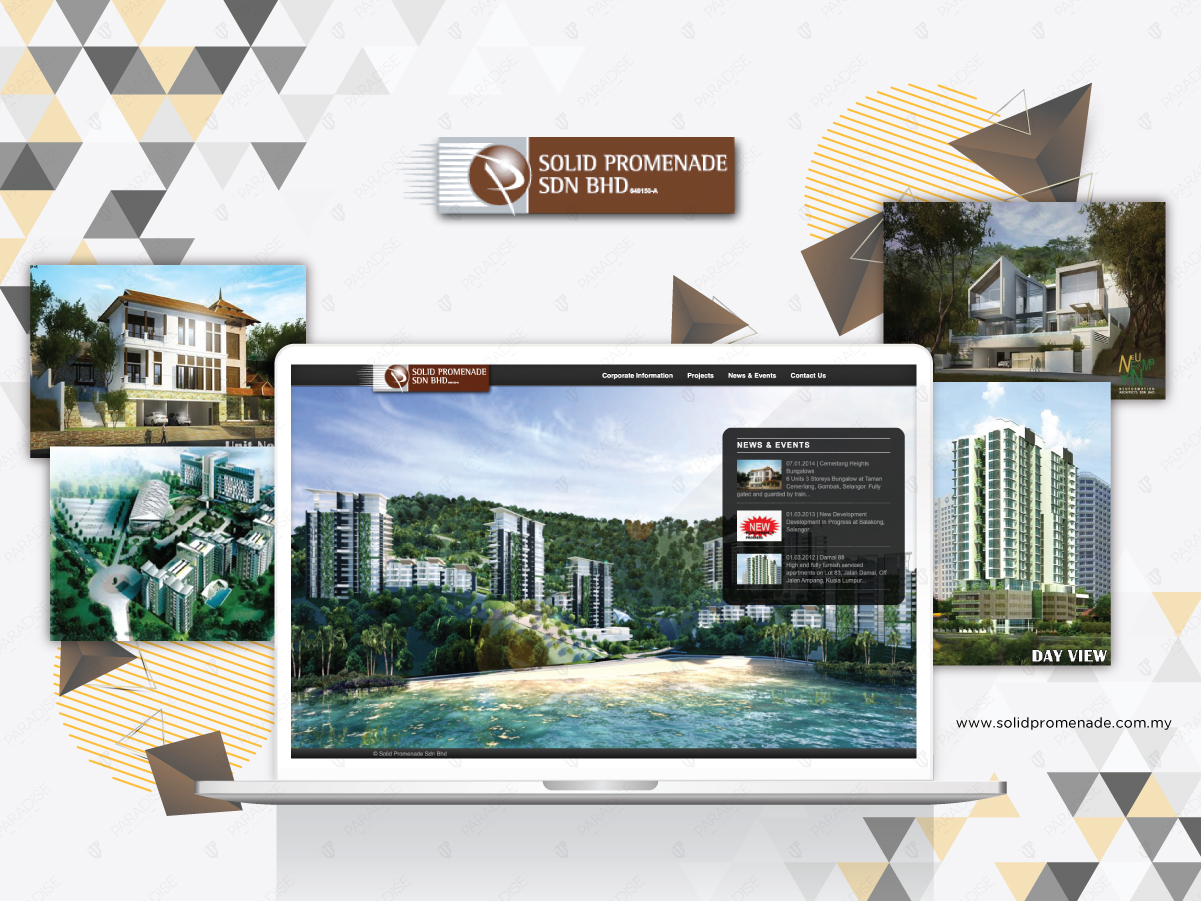The webpage features a prominent banner in a rectangular outline. The left side of the banner is gray and contains a brown circle with an ornate 'D' set against several horizontal gray lines. The right section, extending from the left edge to the end of the box, is brown and displays the text "Solid Promenade SDN BHD" along with some smaller, unreadable text.

Below this banner, there's an image of a computer screen displaying the same "Solid Promenade SDN BHD" label in its top-left corner. The screen features navigational tabs labeled "Corporate Information," "Projects," "News and Events," and "Contact Us." In the main area, a picturesque scene of rolling, green hills dotted with lush trees transitions into a high-rise-laden skyline. In the foreground, a sandy beige beach with palm trees meets turquoise and blue waters.

A pop-up banner titled "News and Events" appears, showing an image of a three-level building, though the text on it is unreadable. Adjacent to this, a white box labeled "New" lists three lines of text beside it. Towards the bottom, another high-rise building is depicted with four lines of text next to it, albeit too blurry to discern, even upon enlargement.

To the left of the computer screen, there are two images: the first is the same three-level house found under "News and Events," and the second showcases luxurious high-rise buildings surrounded by trees and possibly water.

Underneath these images, there are yellow, blue, and brown lines whose significance is unclear. On the right side, there are two more images: a modern two-level building with large windows, flanked by trees against a clear blue sky, and another high-rise building labeled "Day View." The text above this second building suggests a view but remains unreadable.

The website URL "www.solidpromenade.com.my" is displayed, and each corner of the page is adorned with small triangular banners in gold, gray, and white.